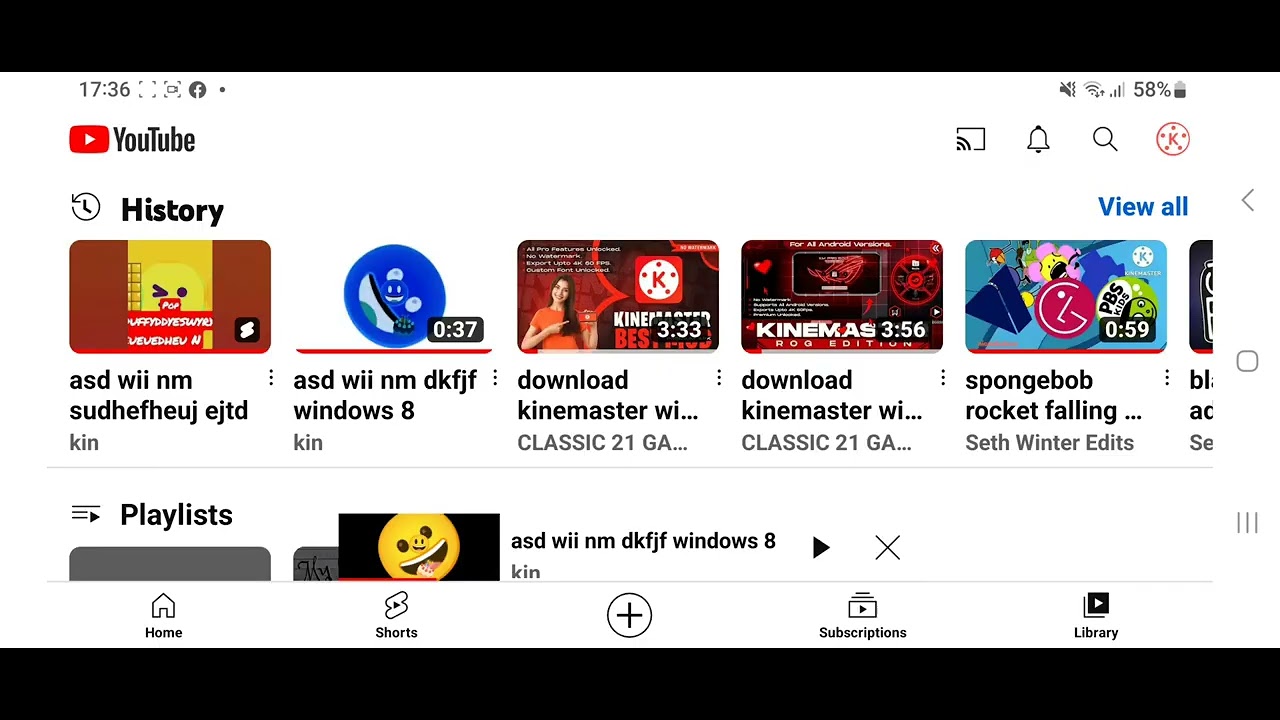The image features a smartphone held in landscape orientation. Displayed on the screen is the YouTube app, with the time visible at the top left corner indicating 17:36. The top right corner shows several status icons: a muted speaker icon, Wi-Fi signal strength, and a battery percentage at 58%. Below these, the YouTube app is open to the 'History' tab, displaying a list of previously watched videos with titles such as "ASD," "Wii," "NM," "Download," "KineMaster," and "Spongebob." Further down, there are various playlists, though one is greyed out and unreadable. The standard YouTube navigation bar is present at the bottom, allowing access to Home, Shorts, video upload options, subscriptions, and the Library. Additionally, just beneath the battery status, there are notification, search, and a mysterious "K" inside a circle icons, further enhancing the interface's busy yet familiar look.